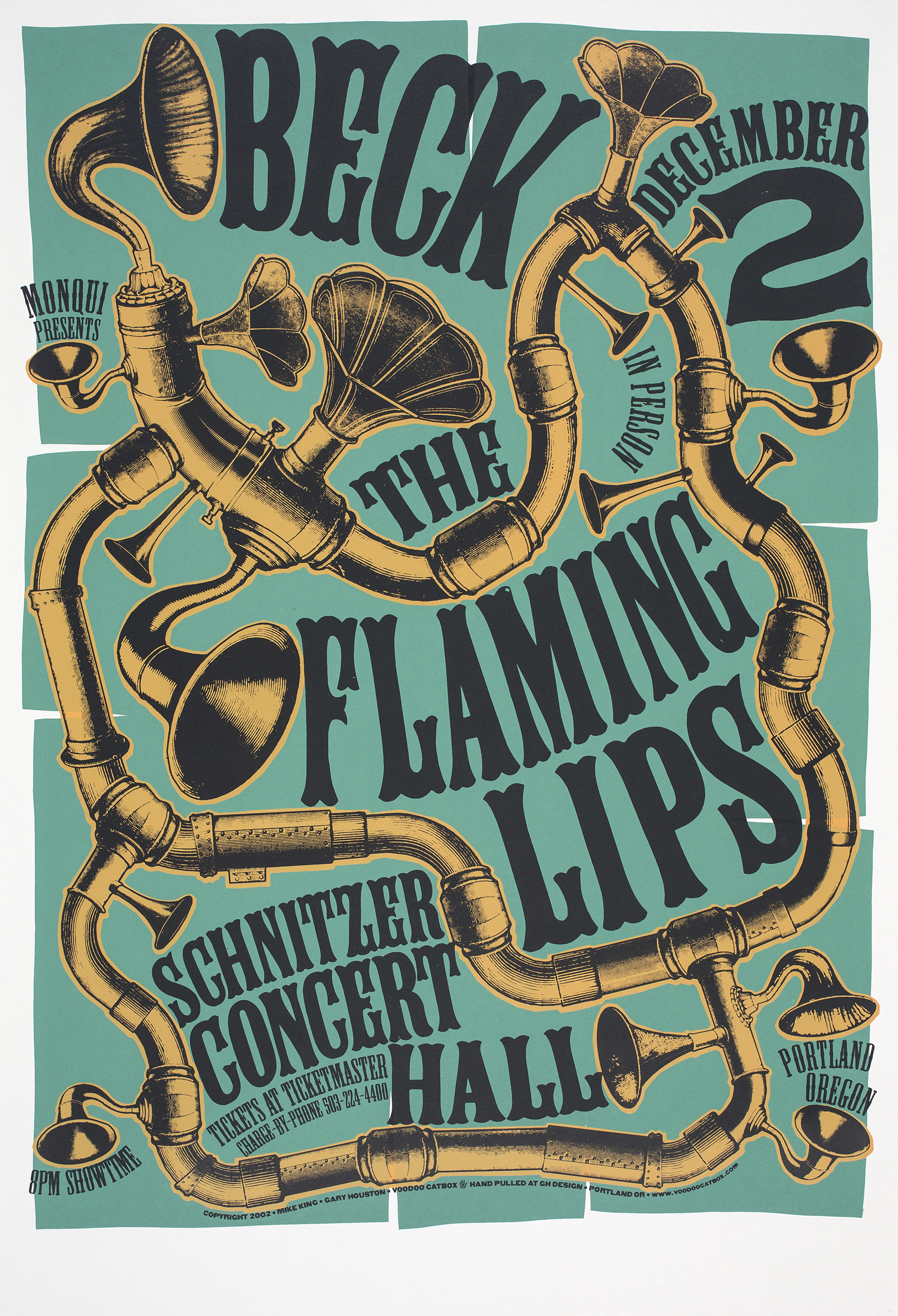This is a detailed concert poster for a show on December 2nd at the Schnitzer Concert Hall in Portland, Oregon, featuring musical acts Beck and The Flaming Lips. The poster, designed in portrait alignment, announces an 8 p.m. showtime with tickets available at Ticketmaster. The intricate design showcases a backdrop of bluish-teal, or seafoam green, segmented with small white gaps. Over this background, a series of interconnected metal pipes forming an intricate network is depicted, out of which numerous mini-megaphones (resembling gramophone horns) emerge. These pipes and megaphones are rendered in a goldish-yellow and black color scheme. The text of the poster, written in dark navy blue, includes additional details: "Mongke presents Beck in person, The Flaming Lips," along with a contact number (503-224-4400) and a copyright notice, "2002 Mike King and Gary Houston, Voodoo Catbox Hand-Pulled GH Design, Portland, Oregon." Further information and designs can be found at www.voodoocatbox.com. This poster blends a vintage gramophone aesthetic with a modern concert announcement, creating a visually captivating advertisement.